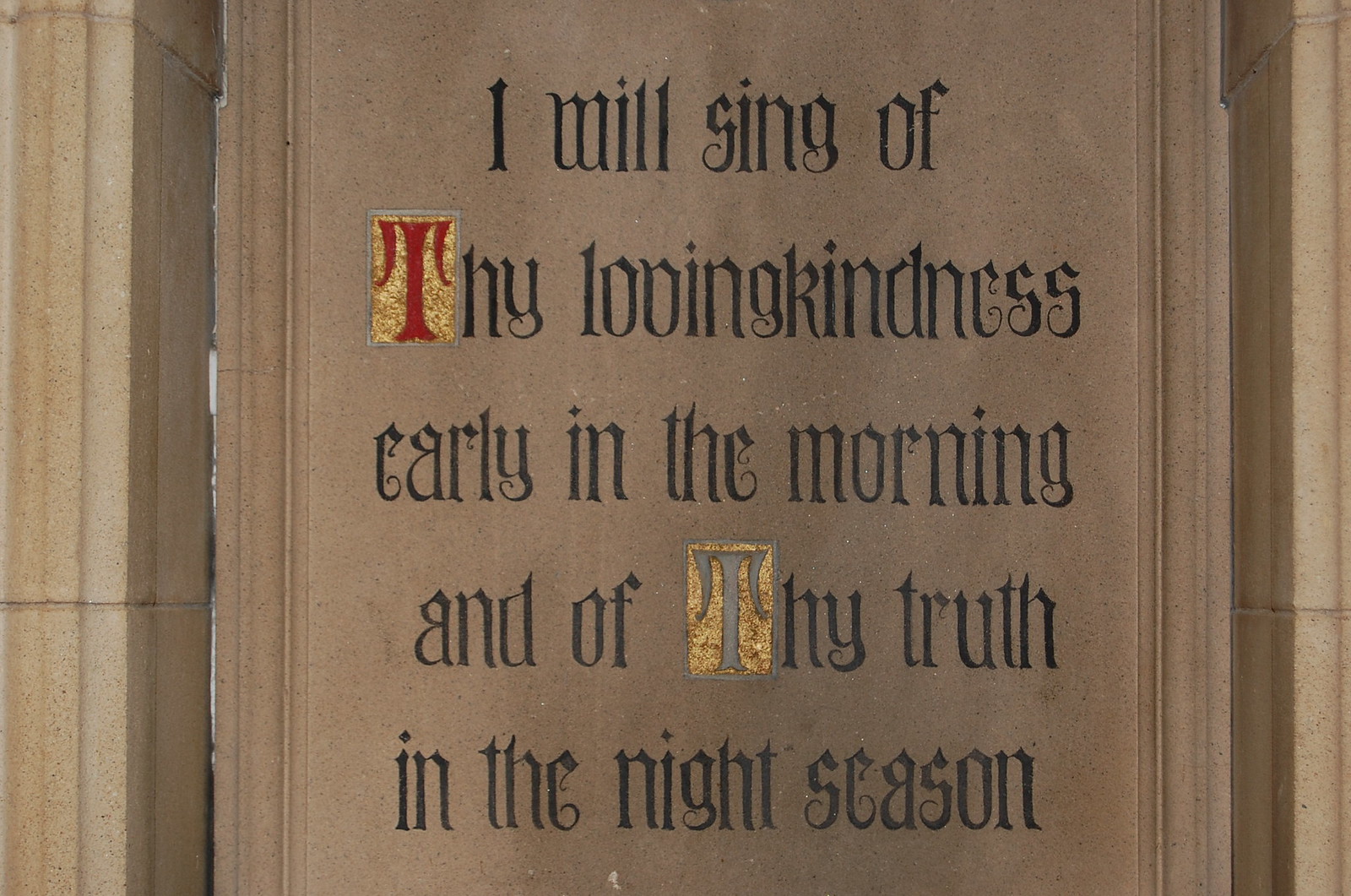This is a detailed picture of a stone wall featuring an inscription in old-fashioned, medieval-style font. The text reads, "I will sing of thy loving kindness early in the morning, and of thy truth in the night season." The letters are primarily black, but notable emphasis is placed on the word "thy" which appears twice. The first "T" in "thy" is in red with a gold background, while the second "thy" has a gray "T" also set against a gold background. The inscription appears to be carved into large cement blocks, with visible seams and grout between them. The image is closely cropped, focusing solely on the text and stone, leaving it unclear whether the location is indoors or outdoors.